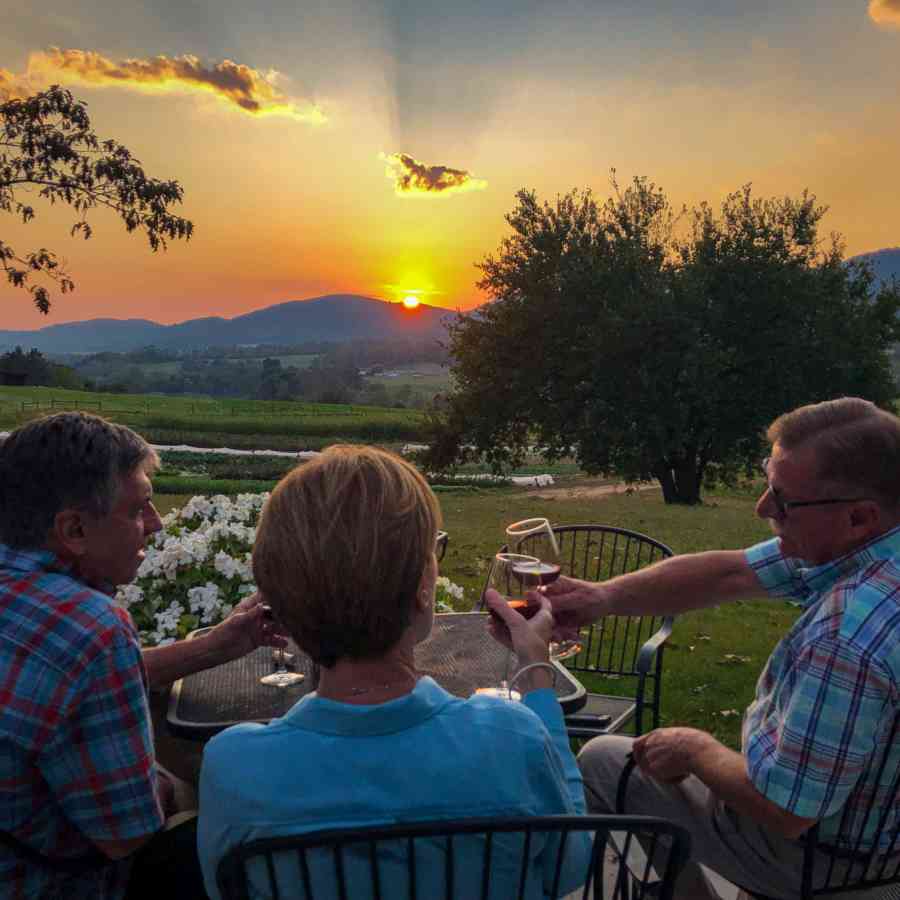The photograph captures a serene moment of three older individuals seated at a square metal table, enjoying a sunset toast with wine glasses filled with a reddish liquid, likely wine or champagne. They are positioned outside in iron wicker chairs, with a scenic backdrop of a golden-yellow sky, lightly colored clouds, and a mountainous horizon. A dark, shadowy tree frames the left side of the image, while another tree appears in the back right. A white-flowered bush adds a touch of nature to the scene. 

In the foreground, a woman with medium-length blondish-brown hair, wearing glasses and a blue shirt, and holding a wine glass in her right hand, is seen over the shoulder. To her right is a man with gray hair parted on the side, donning black glasses, a mustache, and a short-sleeved blue, red, and green plaid shirt paired with gray shorts. On her left sits another man with messy dark gray hair, wearing a blue plaid shirt. The trio is engaged in a cheerful toast as they watch the sun dip below the distant mountains, casting a warm glow over the peaceful, green field before them.